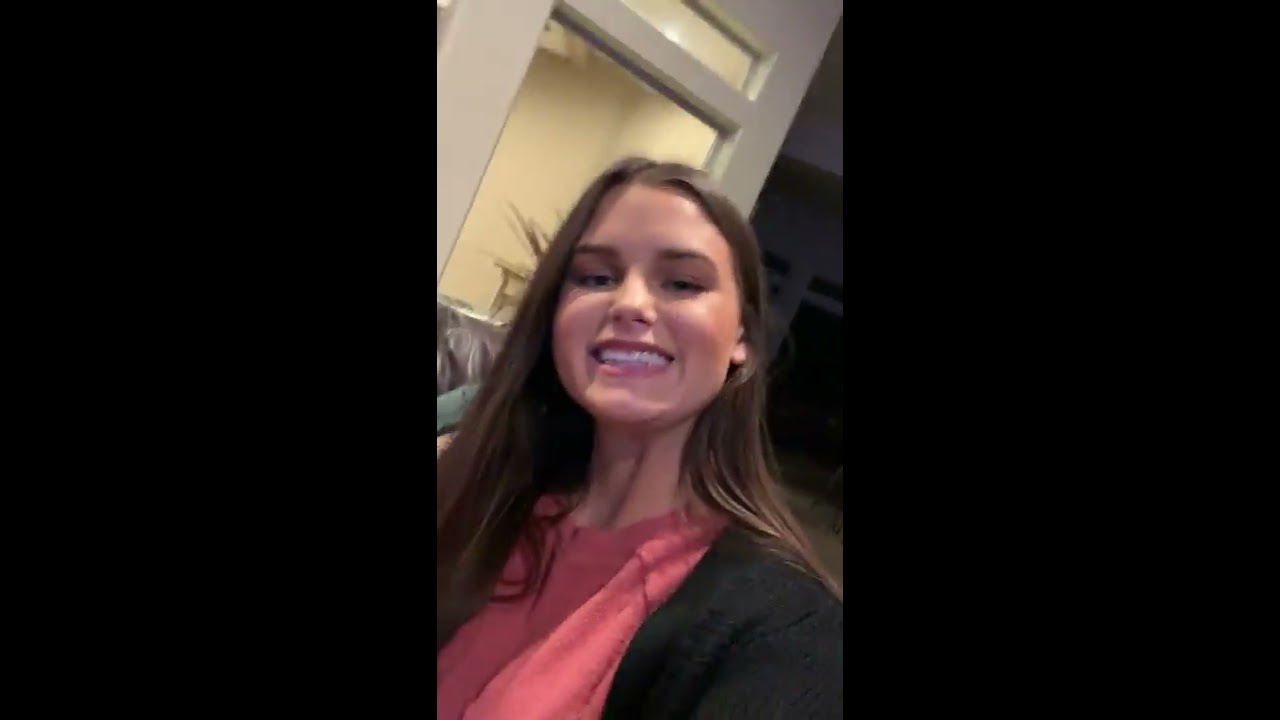The image features a young woman in her twenties with long brown hair, smiling radiantly at the camera. Her big, white-toothed smile is striking and exudes a sense of happiness and contentment. She is wearing a pinkish shirt underneath a black jacket. In the background, there's a dimly lit window, possibly of a house, with a glimpse of a plant visible, although her head covers most of the background details. The picture shows her head slightly tilted back and turned a bit clockwise, with noticeable shadows on her face caused by a bright overhead light, creating a contrast between her illuminated cheek and forehead. The image is framed by large black rectangular borders on both the left and right sides, centering her perfectly in the middle of the shot, with no visible text or inscriptions on her clothing.